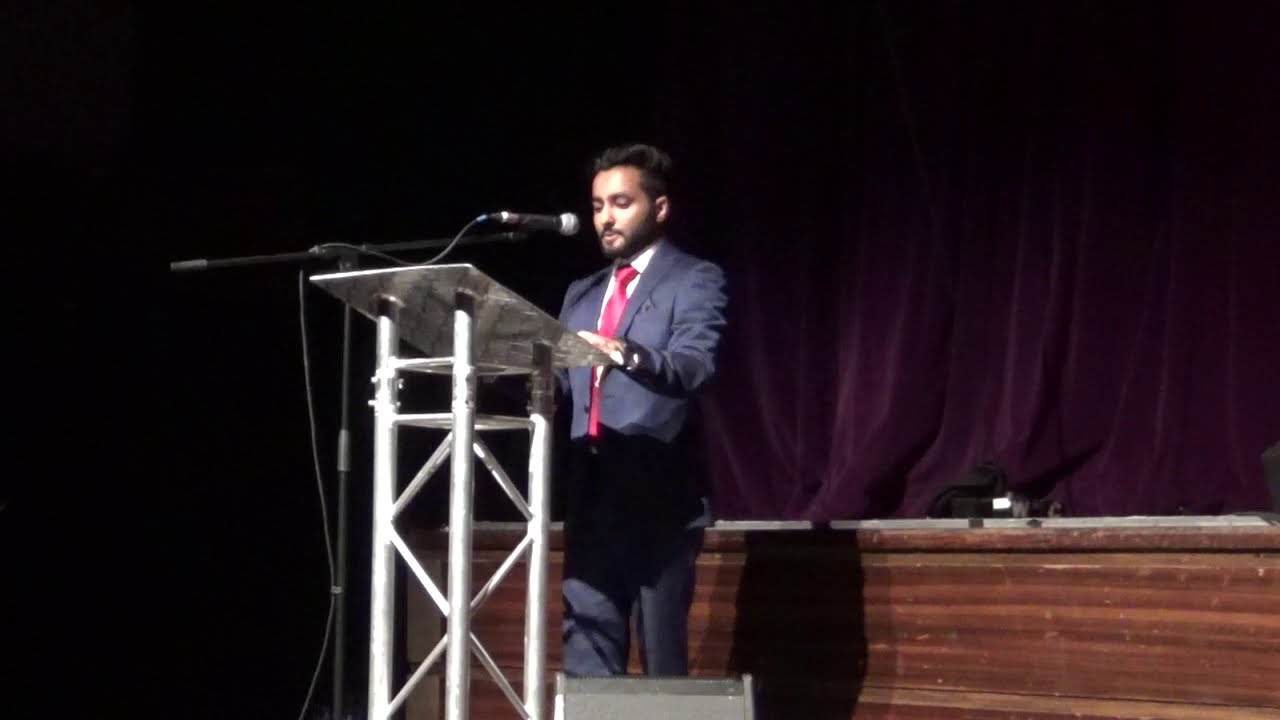In this image, a middle-aged man, who appears to be of Middle Eastern or Indian origin with short dark hair and a trimmed beard, is speaking into a black microphone at a podium. He is dressed in a navy blue suit, complemented by a white shirt and a shiny red tie. The man is positioned on a stage with a podium that has a distinctive metal frame, reminiscent of scaffolding, with a grid-like design and a flat surface that might be glass or metal. He is reading from something placed on this podium, which seems slightly elevated in relation to his height.

The scene behind him is mostly dark, but on his right, there is a distinctive plum-colored curtain that is entirely closed and extends down from a higher stage area. This curtain and the wooden barrier in front of him, made of dark brown wood, enhance the theatrical setting, suggesting he is delivering a speech or a presentation in a large room or auditorium. The background on the left side of the podium fades into darkness, making the man the central focus of the image.